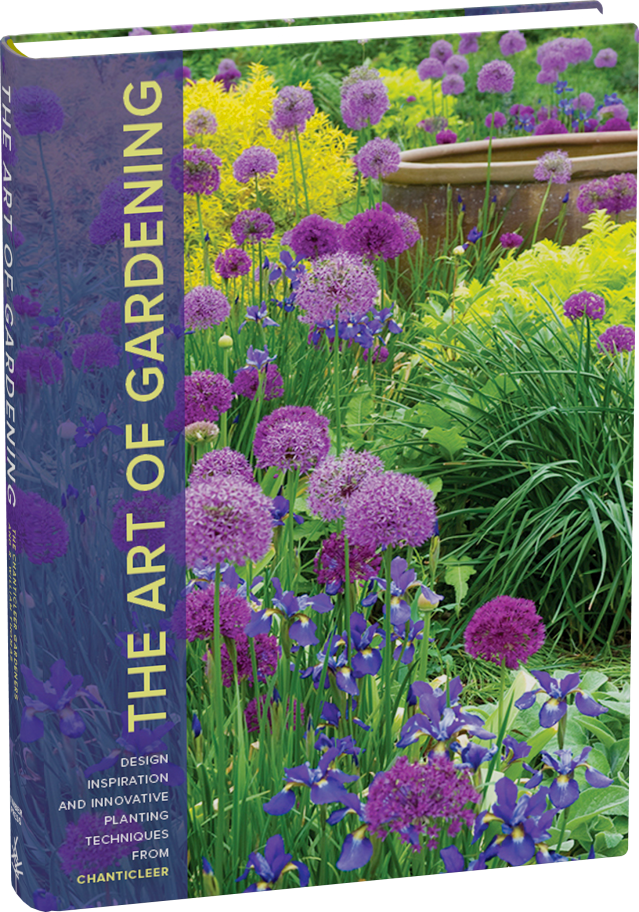The image displays a book titled "The Art of Gardening," with the additional text "Design Inspiration and Innovative Planting Techniques from Chanticleer" shown sideways along the spine. The book is positioned diagonally, leaning toward the bottom left. The cover features a richly detailed garden scene. There are clusters of round, purple flowers in various shades—some dark, some lighter—interspersed with vibrant yellow bushes and lush green grass. Near the upper part of the image, between two bushes, sits a large, round, brown bucket or wooden garden structure. The overall garden display on the cover showcases a variety of colorful plants, emphasizing the book’s theme of innovative gardening techniques.